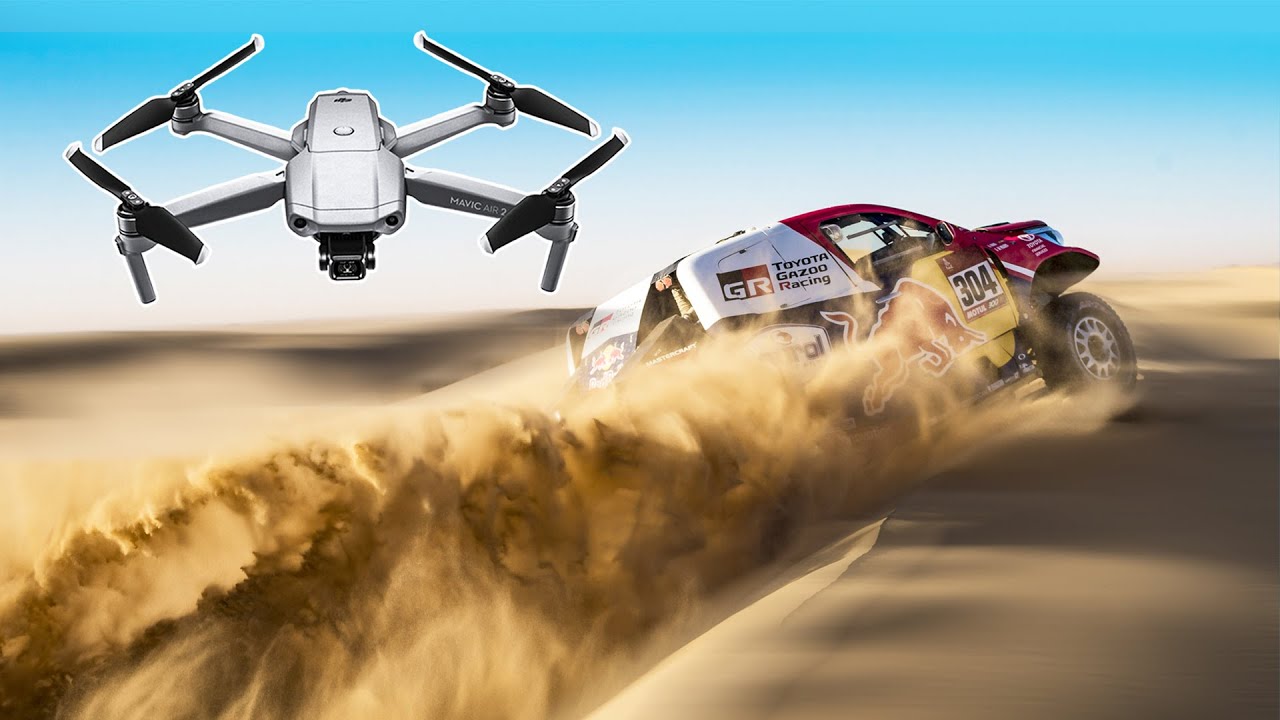In this striking digital artwork, a dynamic scene unfolds in a vast desert filled with brown sand dunes stretching to the horizon. Dominating the scene is a sleek sports car, heavily decorated with vibrant designs and logos, prominently displaying the number 304 and the markings of Toyota Gazoo Racing. The car, painted in a vivid mix of white, red, black, and yellow, is captured mid-motion, leaning slightly to its left with a massive plume of sand billowing in its wake, emphasizing its high speed. In the sky above, a bright blue expanse contrasts with the arid landscape below. Towards the upper left, a four-propeller drone hovers close to the action, presumably capturing stunning aerial footage of the exhilarating race. The drone is predominantly white with black wings, adding a high-tech element to this thrilling desert race scene.